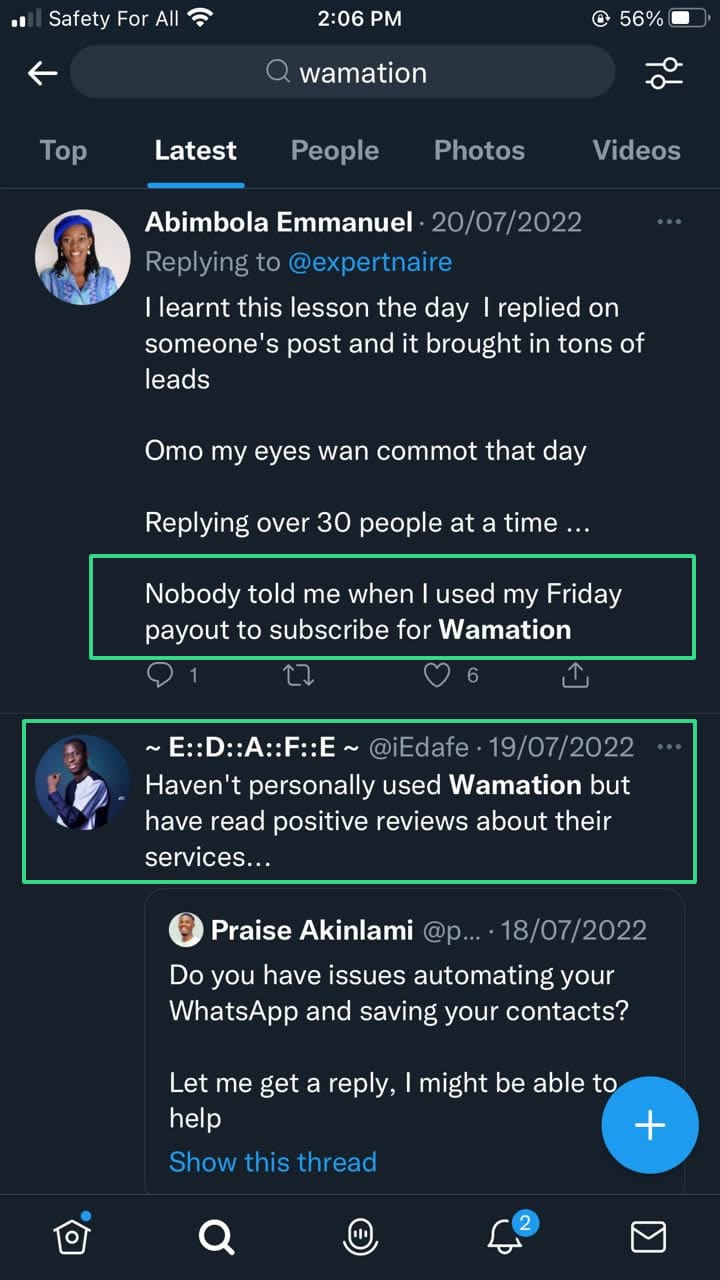The screenshot displays a smartphone screen with a black background. In the top left corner, there are two signal bars adjacent to the phrase "Safety for All," followed by a full Wi-Fi signal icon. At the center of the screen, the time reads 2:06 PM. On the far right, next to an unidentified symbol, the battery level is shown at 56%. 

The user appears to be on the Twitter (now rebranded as X) app. At the top of the screen is a search bar with the term "Whamation" entered. Below the search bar, there are clickable tabs labeled "Top," "Latest," "People," "Photos," and "Video." The user has selected the "Latest" tab.

The first post visible is by Abimbola Emmanuel, stating: "I learned this lesson today. I replied to someone's post, and it brought in tons of leads. Oh my, my eyes won [and] comment that day. Nobody told me when I used my Friday payout to subscribe for Whamation." 

Following that is a post from EDAFE, who is replying to a user named Praise Akilami regarding automating WhatsApp and saving contacts. EDAFE mentions, "I haven't personally used Whamation, but have read positive reviews about their services."